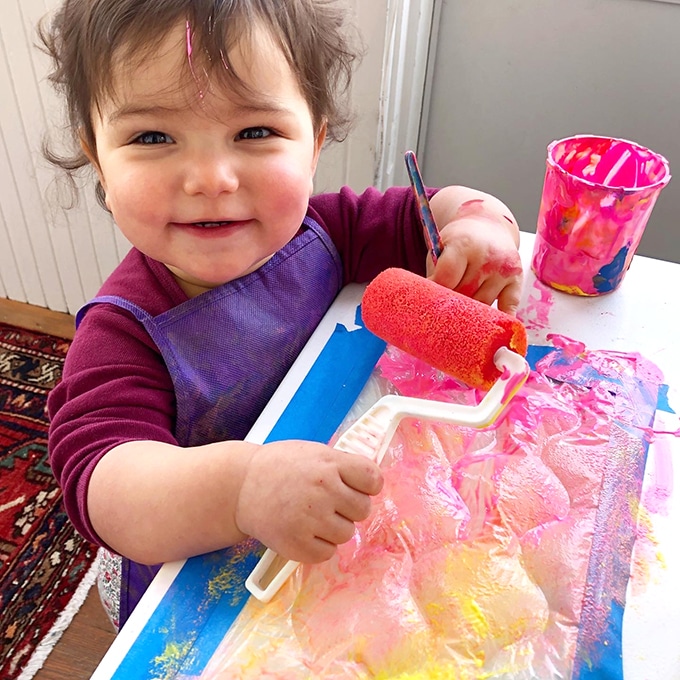This photograph captures a charming scene of a toddler deeply immersed in painting. The toddler, with brown hair streaked with pink paint, is smiling brightly at the camera. She has a roller paintbrush with a red spongy top in her right hand, and her left hand is smudged with pink paint, possibly from holding a small paintbrush. She is wearing a burgundy shirt with the sleeves rolled up, covered by a purple apron. In front of her is a white shelf or table, upon which a piece of paper or mat is taped down, and she is diligently rolling paint onto it. To her left is a cup filled with pink paint. The background includes vertical blinds or a sliding glass door, and a rug with an Aztec-like pattern featuring dark reds and greens. The toddler’s joyful expression and artistic efforts make for an endearing and lively image.